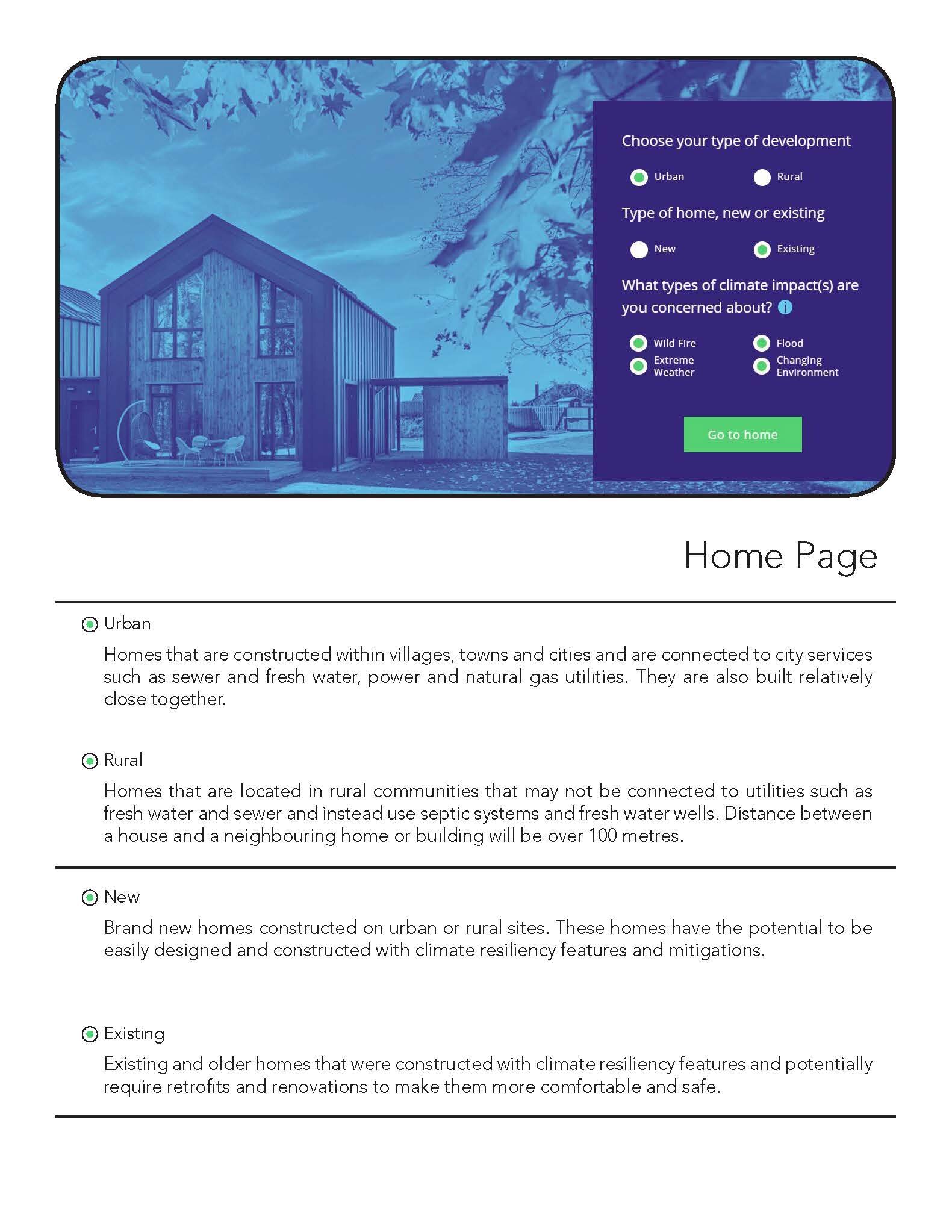**Detailed Caption:**

The image showcases a modern rural hybrid home situated in the serene countryside. The house features a minimalist design fused with contemporary elements, highlighted by a covered porch area on the right side. The foreground is adorned with leaves from nearby trees, adding a touch of nature to the setting. The entire image is rendered in shades of blue, creating a tranquil, duotone aesthetic.

On the right side of the image, there's a comprehensive panel with various options and buttons. The panel is segmented with thin black lines and includes the following selections:

- **Type of Development:**
  - Urban (selected)
  - Rural

- **Type of Home:**
  - New
  - Existing (selected)

Each selected option is marked with a green dot in the middle of a white circle. Users are prompted to select their concerns regarding climate impacts, with the following options highlighted:
  - Wildfire 
  - Extreme Weather 
  - Flood 
  - Change of Environment 

Below these options, a prominent green button invites users to "Go to Home Page." 

Additional informative text details the distinctions between urban and rural homes:

- **Urban Homes:** 
  Homes in villages, towns, and cities connected to city services such as sewer, freshwater, power, and natural gas utilities, built relatively close together.

- **Rural Homes:** 
  Homes located in rural areas that may rely on septic systems and freshwater wells, with distances exceeding 100 meters from neighboring houses.

Furthermore, the panel differentiates between new and existing homes:

- **New Homes:** 
  Brand new constructions on urban or rural sites that can be designed with climate resiliency features.

- **Existing Homes:** 
  Older constructions that may require retrofits and renovations to enhance comfort and safety, integrating climate resiliency features.

This descriptive and detailed caption not only highlights the visual aspects of the image but also encapsulates the informative content presented within the interactive panel.